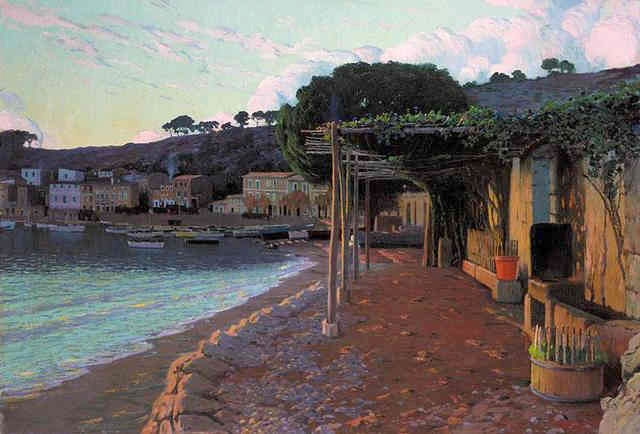This painting depicts a scenic waterfront, where a vibrant blue body of water occupies the left side, suggesting either a river or a seashore. Along the right side, there's a narrow sandy or dirt beach bordered by a small rocky seawall. Adjacent to this shore, a cluster of buildings, predominantly with yellow or light red walls, lends a rustic charm to the scene. Among these structures, the one closest to the viewer features a wooden trellis adorned with lush greenery, possibly a wine plant, wrapping around its yellow walls. 

In the background, a tree-covered hill rises, adding depth and contrast to the composition. The sky above, painted in a delicate light blue, is dotted with soft white and light pink clouds that stretch across the canvas. This artwork captures the essence of an idyllic, possibly European coastal town, with its houses framed by nature and an expansive sky, invoking a sense of peaceful, everyday beauty. The painting is in a landscape orientation, further emphasizing the panoramic view of this serene setting.